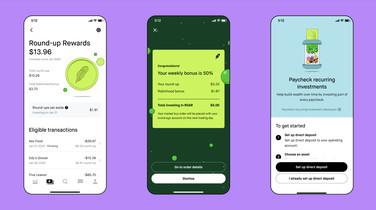The image displays three mobile devices arranged side-by-side on a light purple background, each identical in size and shape. From left to right, the screens of the devices exhibit different displays:

1. **Left Device:** The first device features a white screen filled with numerous small, faint black text and numbers. Dominantly displayed at the top in bold black text is "Round Up Rewards $13.96." Directly below this text, towards the right, there is a light lime green circle.

2. **Middle Device:** The second device shows a black screen with a lime green highlighted rectangular window centrally located. At the bottom of this black screen, a large white button is prominently visible.

3. **Right Device:** The third device's screen transitions from a light blue at the top to a white at the bottom. Positioned at the bottom of the white section, there is a large black button.

Together, the screens likely indicate different stages or interfaces of a mobile application, each distinct in visual design and function.